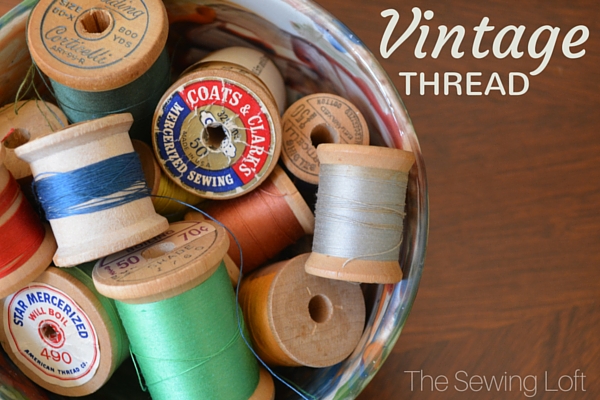The image shows a vintage-themed advertisement featuring a distressed glass bowl filled with various wooden spools of sewing thread, positioned on a wooden table. The shot is taken from an angle slightly above and to the bottom right of the bowl, providing a clear view of the colorful contents. The spools are in a range of colors including dark blue, seafoam green, white, silver, orange, red, and a brighter orange. Each spool appears partially used, with one spool particularly noted for having just a small amount of blue thread remaining. The thread brands visible include "Star Mercerized 490" and "Coats and Clark Mercerized Sewing." The spools are characteristic of vintage sewing kits, complete with the central holes for peg storage. Overlaying the image, the top right corner features the words "VINTAGE" in slight italics and "THREAD" in all caps, while the lower right corner presents the label "The Sewing Loft" in transparent off-white text.